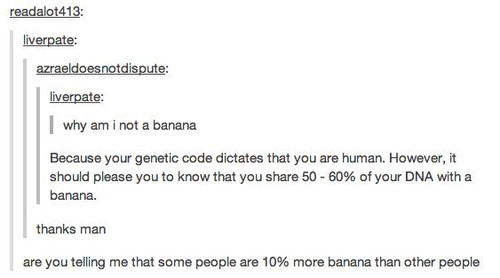The image is a screenshot of a Tumblr post presented like a meme, displaying a humorous conversation on a white background with black text. The exchange begins with "liver pate" asking, "Why am I not a banana?" to which "Azrael does not dispute" responds, "Because your genetic code dictates that you are human. However, it should please you to know that you share 50 to 60 percent of your DNA with a banana." "Liver pate" then replies, "Thanks, man." The conversation concludes with "read a lot 413" humorously questioning, "Are you telling me that some people are 10% more banana than other people?" The text is stacked in chronological order, contributing to the meme's light-hearted tone.